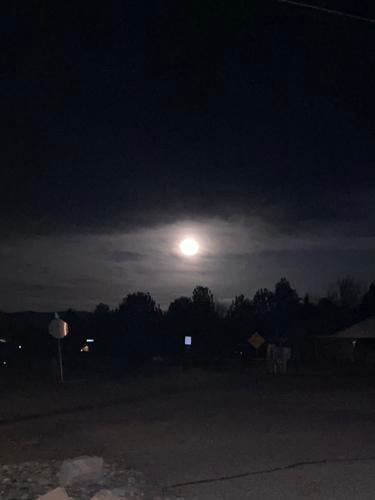A nighttime photograph captures a rural, possibly seldomly trafficked, street scene dominated by a very dark sky taking up the top third of the image. The full moon is centrally positioned but shrouded by a significant layer of clouds, emitting a muted white glow with a hazy aura. Below the sky, a faint tree line stretches horizontally, partially enveloping both the left and right sides of the scene. On the left side of the image, a stop sign, seemingly facing away, is dimly visible near some rocks and patches of grass. Adjacent to this is a concrete object, likely a road feature. Further right, a yellow diamond-shaped street sign subtly stands out. The lower portion of the image hints at a roadway, partially illuminated by unidentified, possibly vehicular, lights reflecting off some of the signs. A building with indistinguishable lighting can be spotted in the backdrop on the right, with the cumulative ambient glow contributing to the ethereal feel of the image.